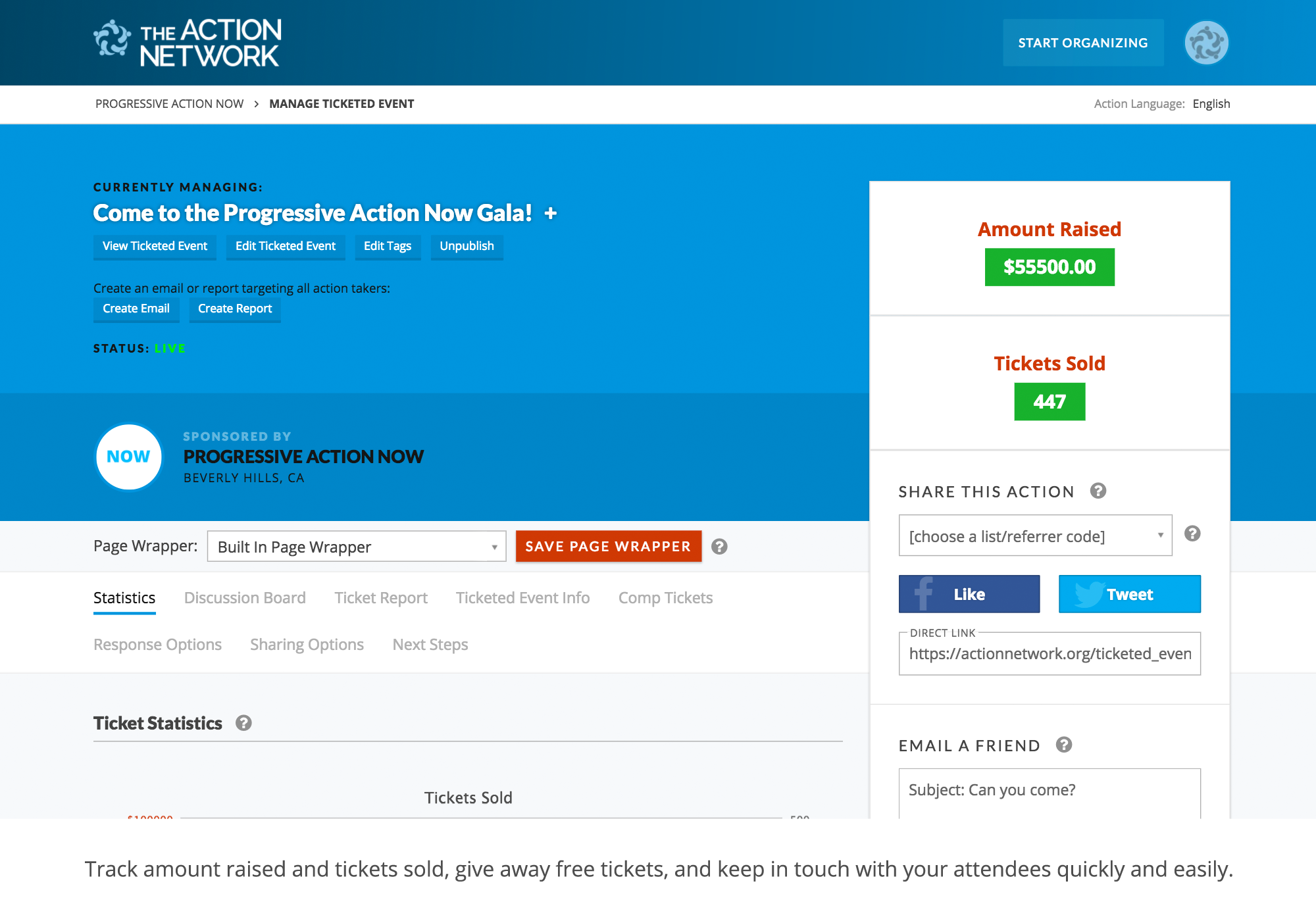The image features a user interface against a blue background, showcasing various interactive elements and a detailed layout.

At the top, a dark blue box contains a swirling blue circle logo, labeled "The Action Network," accompanied by a "Start Organizing" button. Below it, a white box displays the text "Progressive Action Now," accompanied by a right arrow and the option to "Manage Ticketed Event." Adjacent to this is a dropdown menu labeled "Action Language," set to English.

Beneath these elements, a large blue box is segmented into distinct sections. One section reads "Currently Managing: Progressive Action Now Gala," highlighted by a plus mark symbol. Below this header, four buttons are aligned horizontally labeled "View Ticketed Event," "Edit Ticketed Event," "Edit Tags," and "Upgrade."

To the right, the interface provides options to "Create an Email or Report targeting all action takers," along with buttons for "Create Email" and "Create Report." A status indicator at the bottom shows "Live" in green.

On the right side of the layout, a detailed white box includes fundraising information. In red text, "Amount Raised" is shown next to a green button displaying "$55,500." Similarly, "Tickets Sold" in red text is next to another green box showing "447." Additional features include a "Share this action" section with social media buttons for "Like" and "Tweet," a direct link URL, and options to email friends. 

At the bottom of the right panel, tools for event management are listed, such as "Track Amount Raised and Tickets Sold," "Give Away Free Tickets," and "Keep in touch with your attendees quickly and easily."

The footer notes that the event is "Sponsored by Progressive Action Now, Beverly Hills, California," featuring a "Now" indicator marked in blue within a circle.